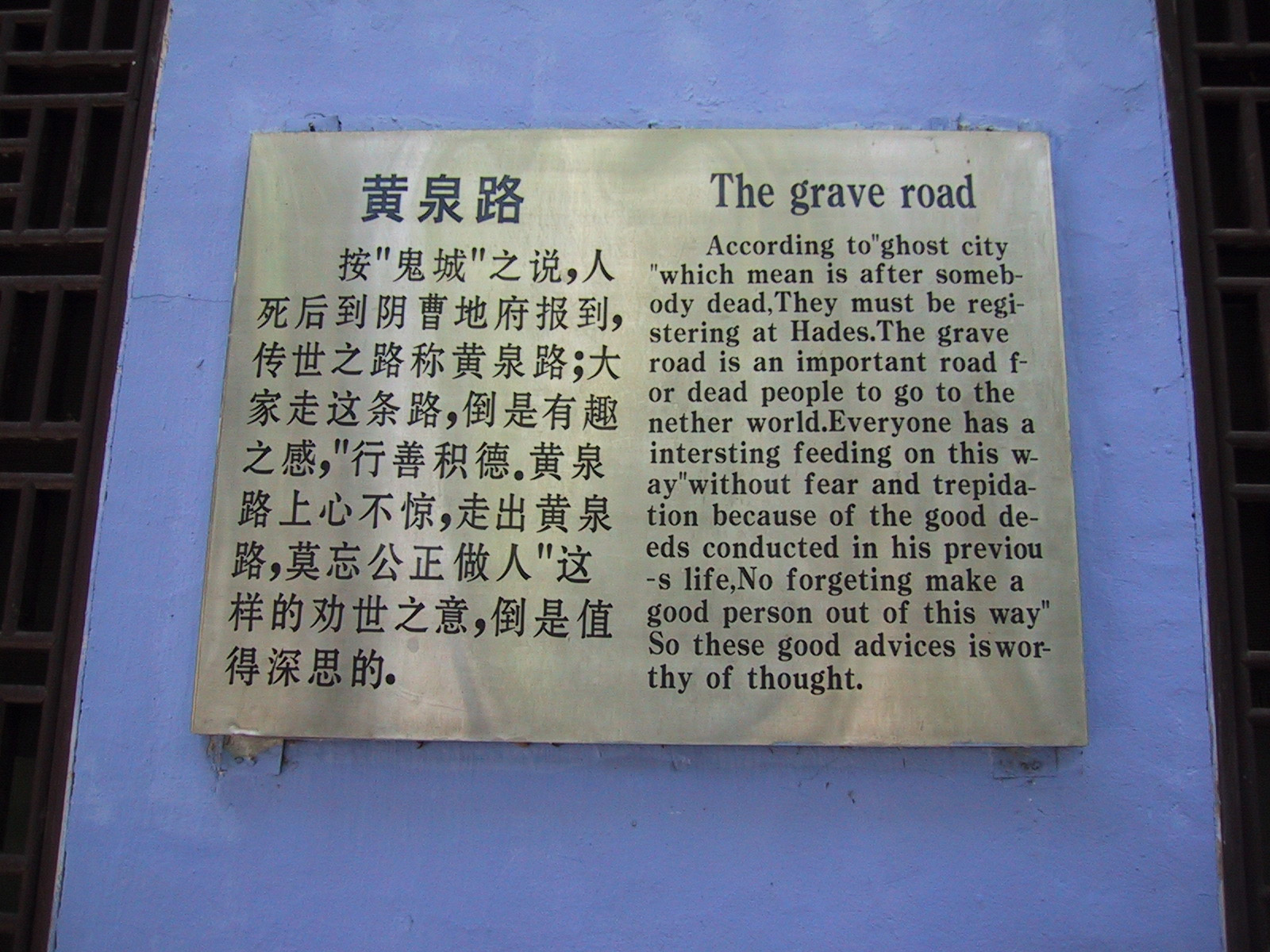The image features a blue background with what appears to be a plaque prominently displayed in front of it. The plaque contains a combination of black and blue text, with the text primarily written in an Asian script, featuring rows of intricate symbols. The layout of the text is symmetrical, with a large, prominent font centered on the left side, followed by nine more rows beneath it. The plaque is encased within a rectangular frame, resembling a structure or holder made of metal bars.

To the right of the Asian script, there is an English translation that reads: "The grave road according to ghost city which means, after somebody dies, they must register at Hades. The grave road is an important path for the deceased to take to the netherworld. Everyone is encouraged to walk this path without fear because of the good deeds conducted in their previous life. It is a reminder to live a righteous life to ensure a peaceful journey in the afterlife. These wise words are worthy of reflection."

This detailed caption provides a comprehensive description of the image, highlighting the visual elements and conveying the cultural significance of the text on the plaque.